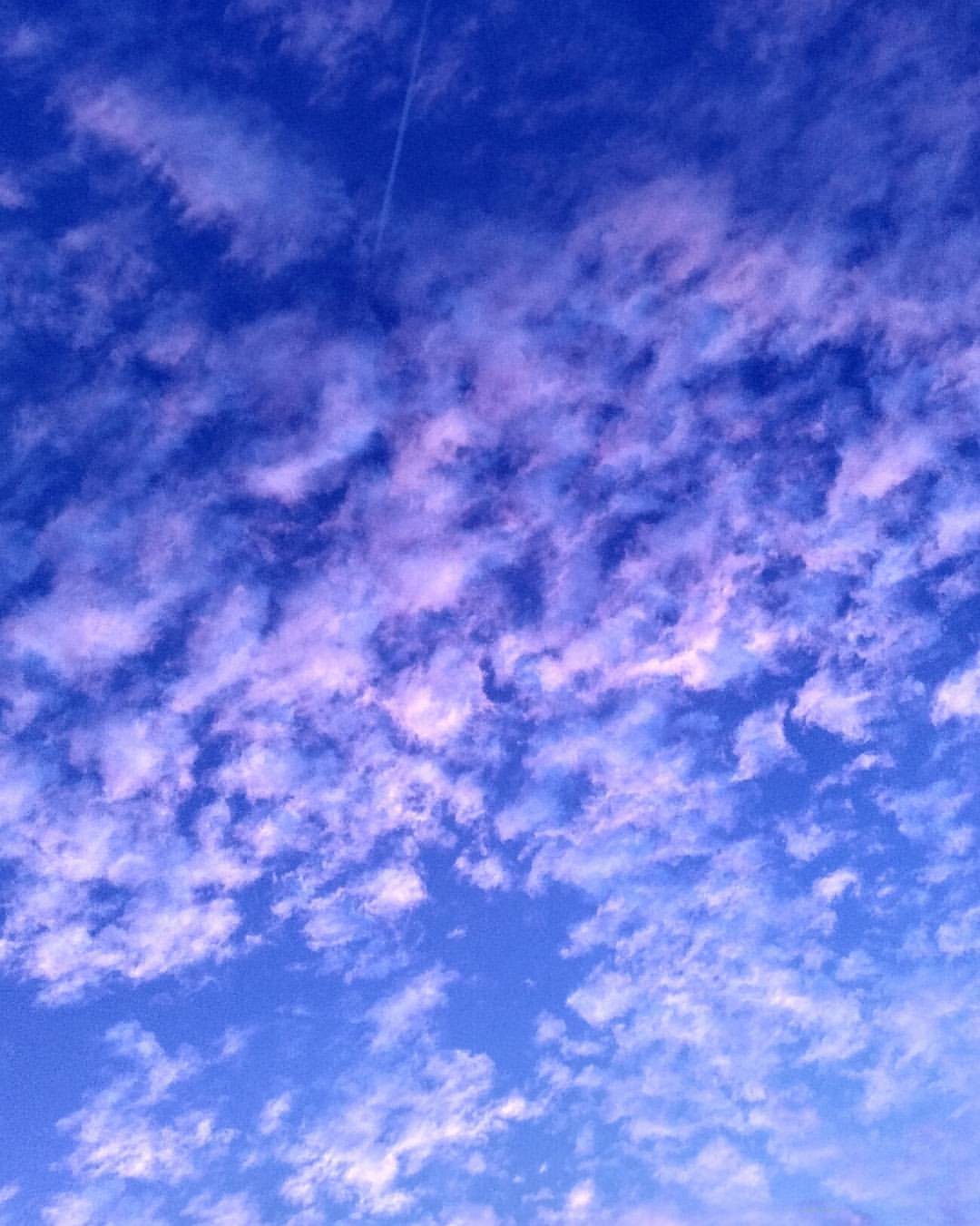The image is a vertical photograph showcasing a stunning outdoor sky scene. The gradient of the blue sky transitions from a lighter shade at the bottom to a darker, almost purplish blue at the top. Scattered clouds are present throughout the image, with more sparsely spread, lighter-colored clouds at the bottom, gradually becoming denser and more vibrant, with hints of pinkish hues, as they ascend towards the top. Amidst the clouds at the upper center, a distinct contrail from a jet cuts a straight line through the sky, adding a unique element to the otherwise organic forms of the clouds. This image, devoid of any other objects or text, creates an abstract, almost pattern-like effect as it focuses purely on the sky, evoking a sense of oblivious perspective.